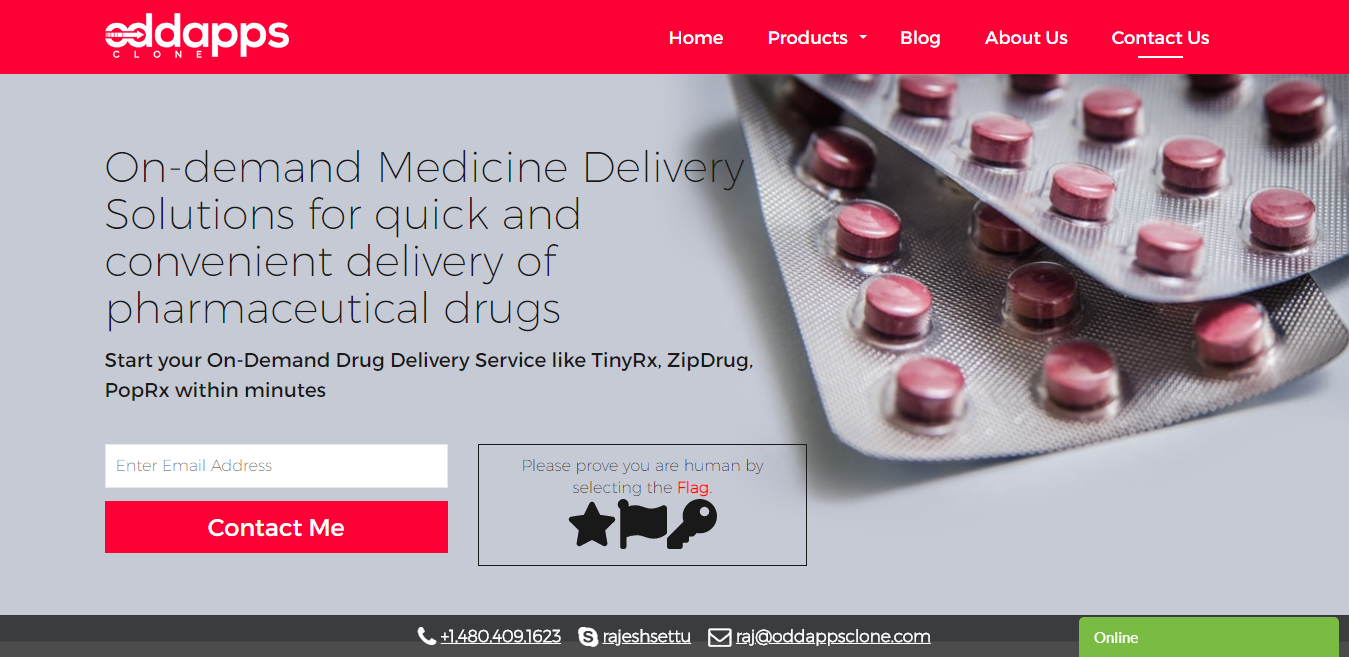The image is a promotional printout from "Odd Apps Clone," showcasing their prescription drug delivery service. The left side of the page features a clickable menu with options for Home, Products, Blog, About Us, and Contact Us, with Contact Us currently selected.

The main focus of the advertisement is on their "On Demand Medicine Delivery" service. The text highlights "Solutions for Quick and Convenient Delivery of Pharmaceutical Drugs" and encourages users to "Start your On Demand Drug Delivery Service like TinyRx, Zip Drug, PopRx within minutes." Below this, there is a field to enter an email address, accompanied by a red "Contact Me" button.

A human verification prompt asks users to prove they are human by selecting a black icon, with options being a star, a flag, and a key. The visual portion also includes two packets of small red prescription pills in silver packaging, emphasizing the pharmaceutical aspect of the service. 

The marketing piece is designed with a gray background and a red border at the top. At the bottom, a black border contains the contact information: "1-480-409-1623, Rajesh Suti," and an email address "Raj@adaptsclone.com." There's also a green tab in the far bottom right corner indicating the service is "online," printed in white text.